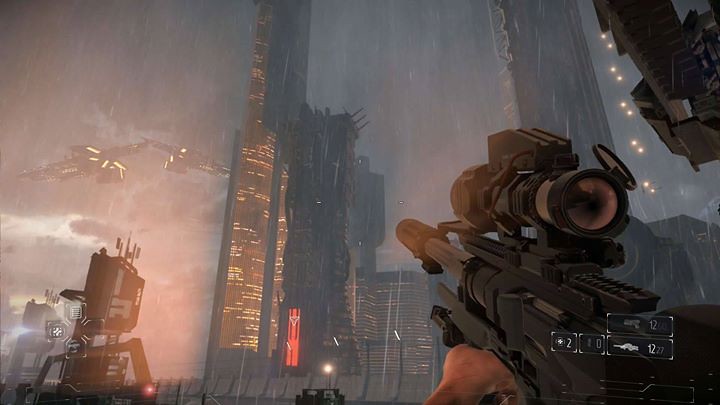This screenshot appears to be from a computer or video game, capturing a player's first-person perspective. In the bottom right corner, the player is holding a large, futuristic machine gun equipped with a scope and a silencer. The player's hand is visibly gripping the trigger. The backdrop of the scene showcases a stormy, dark, and heavily clouded sky, giving an ominous atmosphere. The environment looks futuristic, with towering, illuminated buildings that extend beyond the frame of the image. Two aircraft are seen flying close to the buildings, suggesting imminent action or a mission objective. Overall, the image conveys a tense and immersive experience in a dystopian setting.